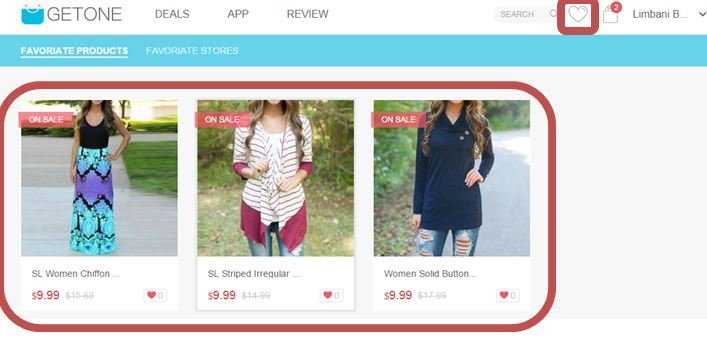A detailed screenshot from the "Get One" online store website is displayed. The interface features dark grayish-black text against a white background, offering a clean and minimalistic design. At the top, prominently positioned, is the store's name "Get One" accompanied by a cyan blue purse icon. The navigation bar spans from left to right, featuring various options: "Deals" for special offers, an app download section labeled "App," and a "Review" section for customer feedback. Towards the right, the navigation includes a search bar for product queries, a heart icon for saving favorites, a notifications icon, and a shopping cart for current purchases. Adjacent to the cart is the user profile section with a dropdown menu for account settings.

Immediately below the navigation bar, a cyan blue menu header highlights sections for "Favorite Products" and "Favorite Stores." The core content area showcases images of merchandise available for purchase. Featured items include:
1. A stylish blue and purple skirt paired with a black top.
2. An eye-catching red and white cardigan matched with jeans.
3. A trendy navy blue tunic-style top accompanied by distressed jeans.

Each clothing item is priced at $9.99 and has been marked as liked by the user, indicating their popularity or interest. The overall layout is user-friendly and visually appealing, making online shopping convenient and enjoyable.